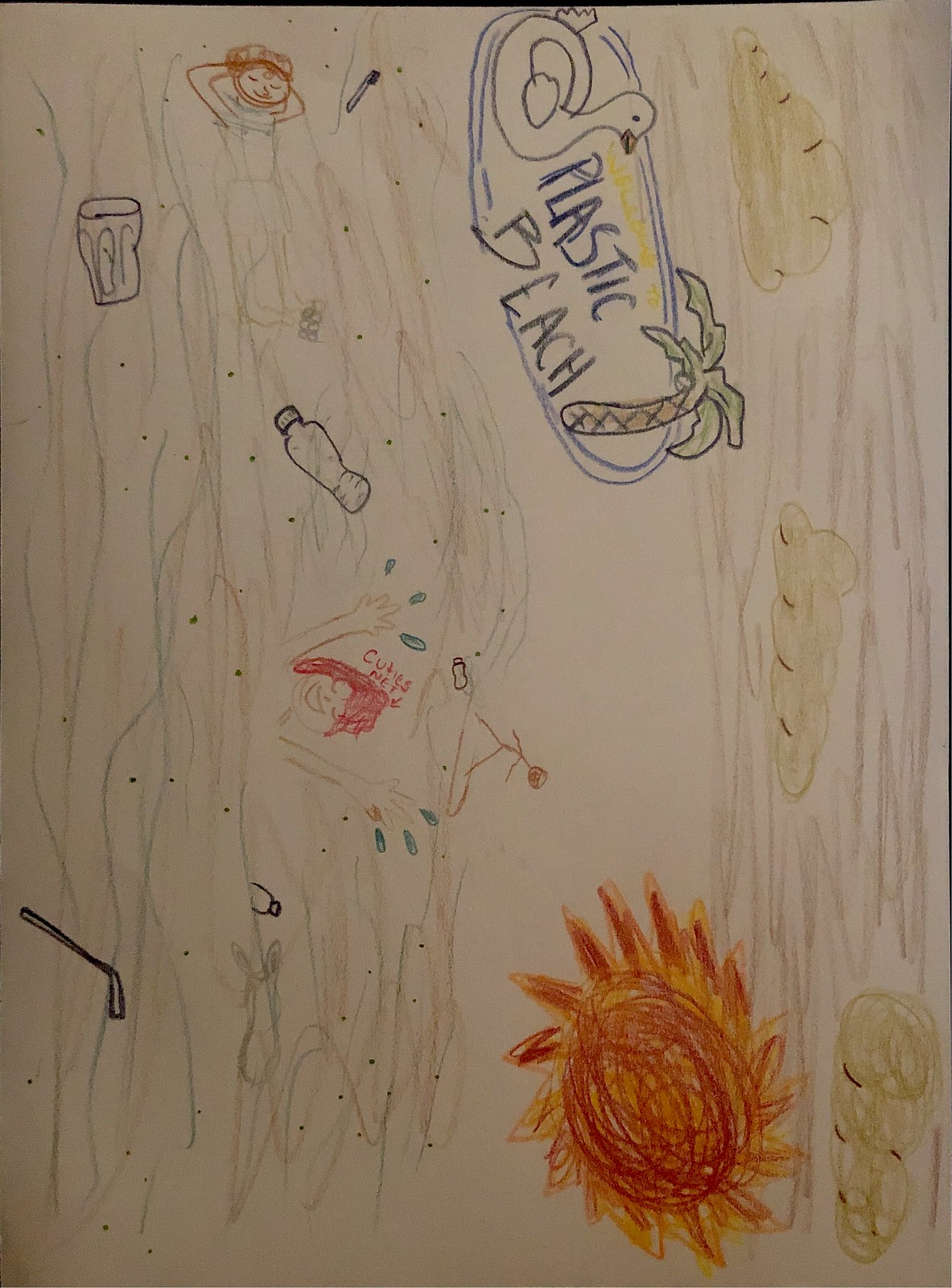In this hand-drawn artwork created on white paper, likely using crayons or colored pencils, the scene depicted is both detailed and evocative. The image is oriented sideways, enhancing its unique perspective. At the top, the sky is filled with brown lines and scattered clouds that also bear brown hues, suggesting a possibly polluted or eerie atmosphere. 

Below these elements lies a strikingly detailed duck, positioned centrally near a small pond area. Next to the duck, the words "Plastic Beach" are inscribed, hinting at an environmental theme. A lone palm tree stands nearby, juxtaposing the natural with the polluted. An orange and yellow sun hovers above, casting a mix of warmth and stark contrast onto the scene below.

The body of water depicted beneath the sun appears significantly dirty, cluttered with various types of garbage that underscore the environmental message of the drawing. Within this polluted water, two figures can be seen swimming, adding a somber, yet oddly hopeful, human element to the piece. The overall composition powerfully reflects themes of pollution, nature, and human impact on the environment.